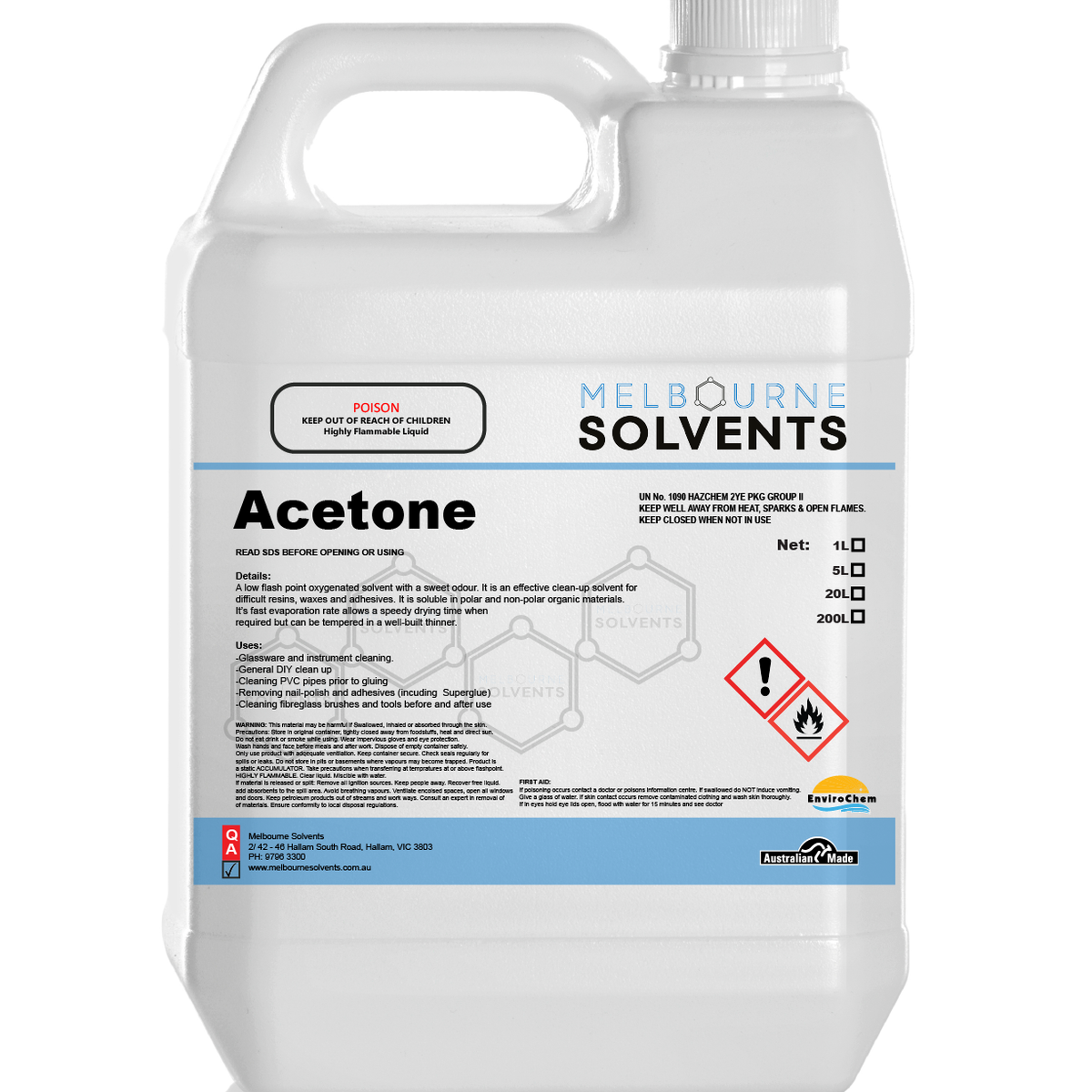The image depicts a large, sealed white container of acetone solvent with a built-in handle and a removable cap at the top. The label on the container is detailed and colorful, primarily featuring blue, red, and black text. It prominently displays the brand name "Melbourne Solvents" in blue and black letters, and it has a significant warning section in red letters that reads "Poison - Keep Out of Reach of Children - Highly Flammable Liquid." There are also warning icons with a red border: one is an exclamation mark and the other is a black flame. The front of the container also includes detailed product information: “Acetone - Read SDS before opening or using,” followed by a description of its properties and uses. The text specifies that acetone is a low flash point, oxygenated solvent with a sweet odor, effective for cleaning difficult resins, waxes, and adhesives. It is soluble in both polar and nonpolar organic materials and has a fast evaporation rate for quick drying. Recommended uses include glassware and instrument cleaning, general DIY cleanup, cleaning PVC pipes prior to gluing, nail polish and adhesive removal, and cleaning fiberglass brushes and tools. The bottom of the label features the "Australian Made" logo and reiterates "Melbourne Solvents." The detailed descriptions and warnings underline its industrial and hazardous nature.